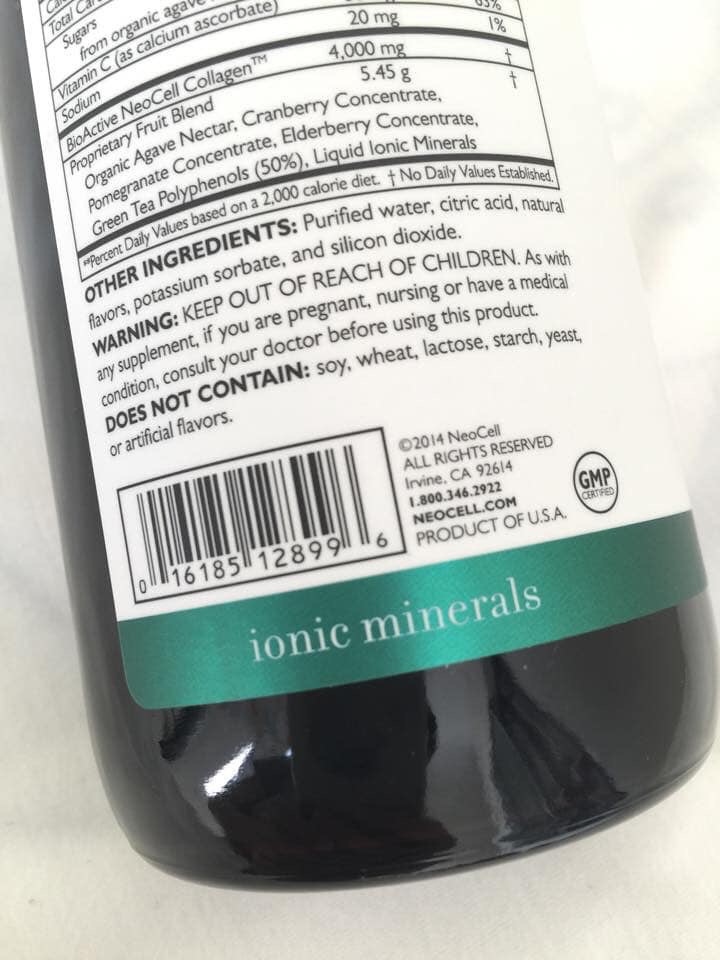The image displays a section of a nutrition label affixed to the back of a black or dark brown glass bottle with a predominantly white label featuring a glossy green banner at the bottom reading "Ionic Minerals." Set against an off-white background, the label includes detailed text in grayish-black lettering. Above the green stripe, key ingredients are listed, such as bioactive Neo-Cell collagen, a proprietary fruit blend, agave nectar, cranberry and elderberry concentrates, pomegranate, green tea polyphenols, and liquid ionic minerals. Additional ingredients mentioned are purified water, citric acid, natural flavors, potassium sorbate, and silicon dioxide. Notably, the product does not contain soy, wheat, lactose, starch, yeast, or artificial flavors. The label includes a barcode, a copyright notice from 2014 by NeoCell, their Irvine, California address (92614), a phone number, and the website neocell.com. Furthermore, the product is GMP certified, indicated by a circular stamp. The warning section advises keeping the product out of reach of children and consulting a doctor if pregnant, nursing, or dealing with a medical condition.